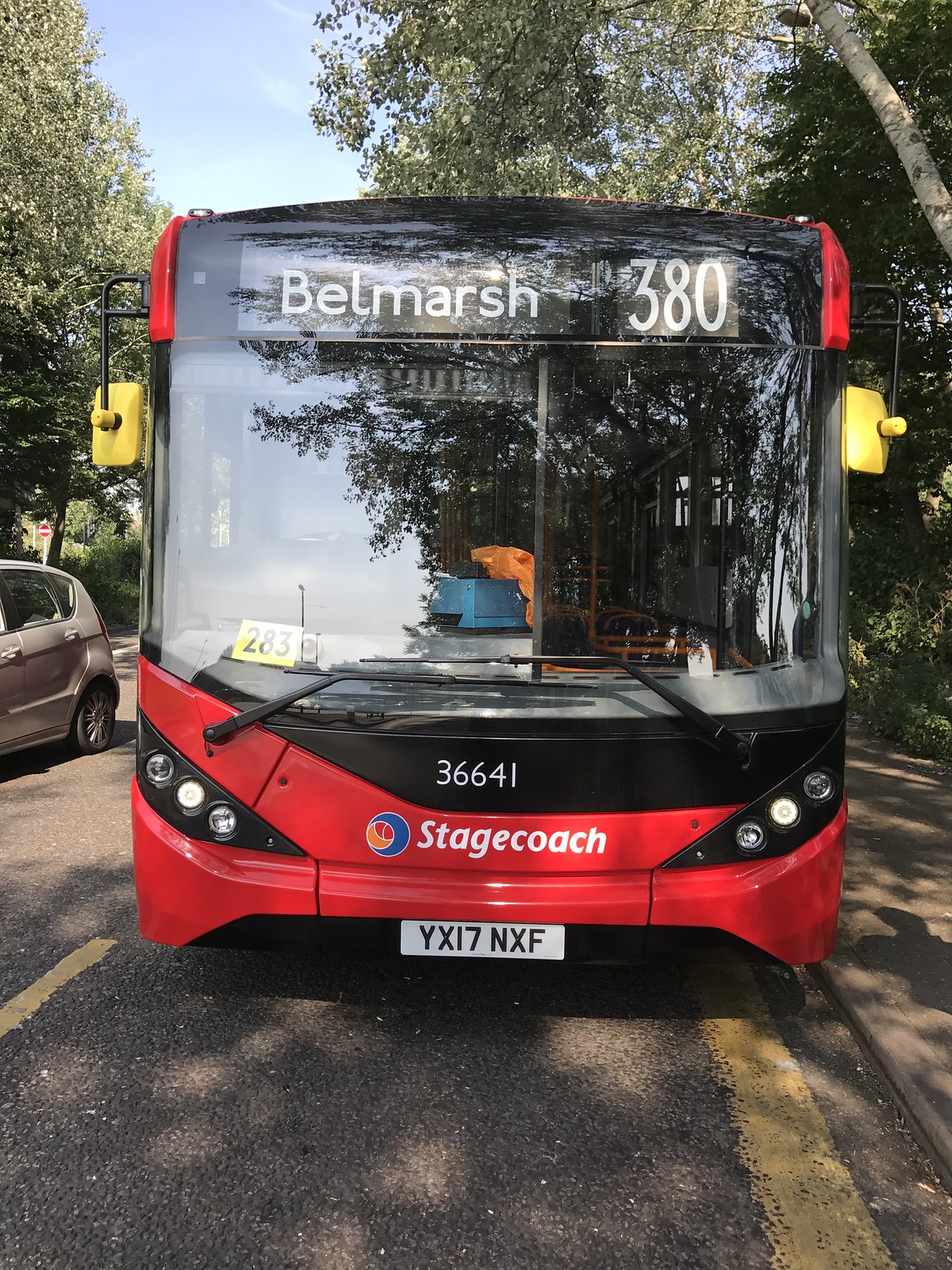The photograph depicts a large, red and black bus with yellow rearview mirrors parked on the left side of a street, likely somewhere in Europe indicated by the license plate "YX17NXF". Above the license plate is the label "Stagecoach" alongside a blue, orange, and red icon. The front of the bus prominently displays "36641" in white on a black panel, and the destination "Belmarsh 380" is shown at the top in white font, suggesting it is part of a dynamically changeable display system. The bus’s front windows are large, and there are noticeable yellow mirrors on both sides. Behind the bus, leafy trees, some flowering white, suggest a spring day. A silver SUV is passing by to the left, and a sidewalk runs parallel to the street on the right. The road features yellow lines, including a broken one to the left of the bus. The image captures the bus primarily in focus with additional details including orange and blue elements inside the bus and a yield sign visible in the background.